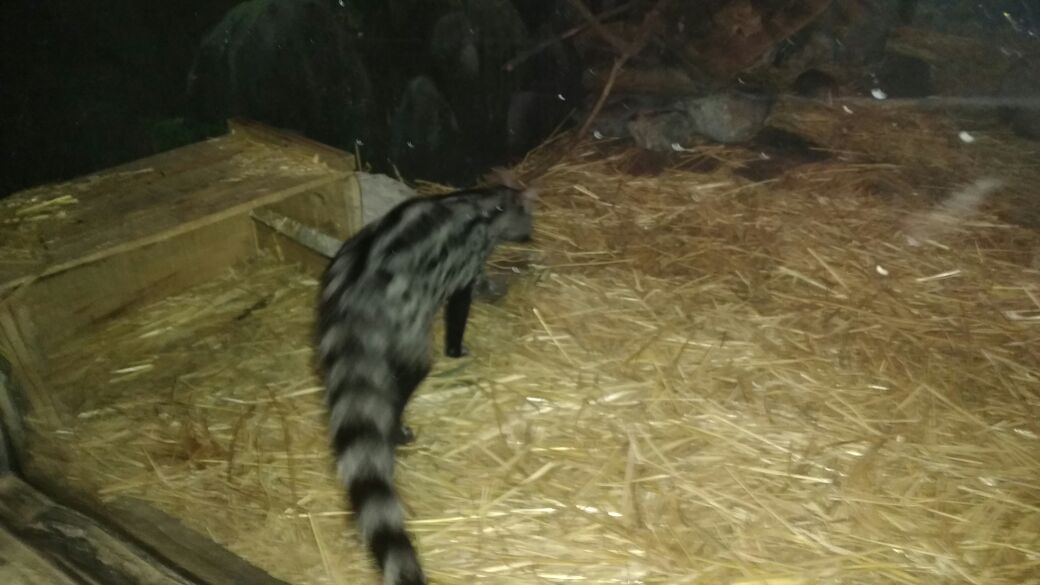This photograph depicts an animal exhibit taken through a plexiglass screen. The image shows an enclosure covered with tan straw scattered on the ground. Just left of center, the back of a mysterious, cat-like animal is visible. The animal has fluffy, black and gray fur with a distinctive long tail adorned with black and gray stripes. The creature is walking away from the viewer, leaving only its back and striped tail extending towards the bottom of the frame. To the left of the animal, there is a wooden box that likely serves as a shelter, while the background reveals a wall designed to look like rocks. The overall setting is somewhat blurry, and the dark background gradually turns reddish towards the right side of the image. The animal's black legs are noticeable, yet its exact species remains unclear, with some comparing it to a skunk, possum, or an oversized rat.